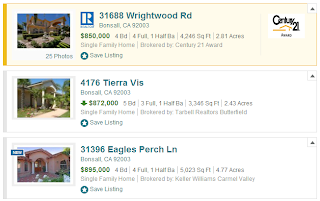The image depicts a small, slightly blurry screenshot of an online real estate listing. The listings are arranged in three rows, each showcasing different properties available for purchase.

At the very top is the first listing, which stands out with its yellow background. This particular element may have been the reason the screenshot was taken. The listing is by Century 21, as indicated in the upper right-hand corner. This listing features a property located at 31688 Wrightwood Road in possibly Bonsai, California, priced at $850,000. It is described as a single-family home. Additionally, there is a note under the image on the left side stating there are "25 photos," although this text is quite difficult to read.

The second row lists a home at 4176 Tierra Vista in Bonsai, California, with a price tag of $872,000. This listing also has a corresponding image on its left side, but fewer details are discernible from the text under it.

The third row features a property on 31396 Eagles Perch Lane, priced at $895,000. Notably, there is a "new" label on the top left corner of the corresponding image, highlighting it as a recent addition to the listings.

Each row ends with an up arrow, likely serving as a navigation button, but its exact function remains unclear. The image's resolution makes some text hard to read, adding to the challenge of getting complete details of the listings.